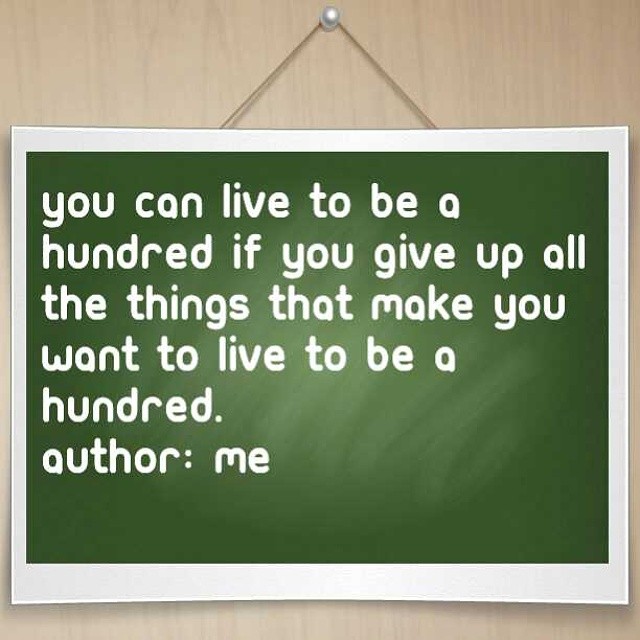The image displays a graphic resembling a framed chalkboard, centrally positioned against a light wood background. A silver metallic push pin at the top center appears to be holding the string attached to the chalkboard frame. The border of this chalkboard is white, and the chalkboard itself is a dark green hue with visible eraser marks, giving it a dusty appearance. The text on the chalkboard is bold and white, reading: "You can live to be a hundred if you give up all the things that make you want to live to be a hundred. Author, me." The design elements emphasize a minimalist yet robust presentation, featuring neutral tones such as beige for the surrounding area and green, white, and blue for the main content.